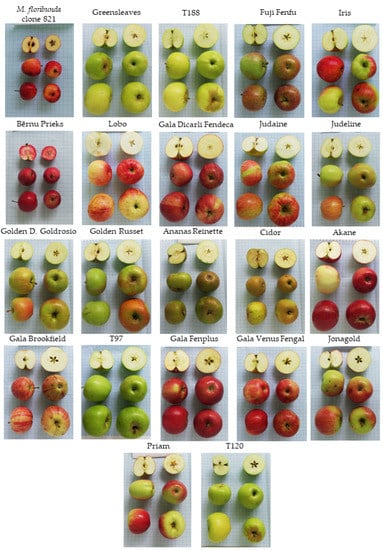This detailed collage showcases a collection of 22 different types of apples, meticulously organized within separate boxes. Each type has its distinct small box, containing six examples of the apple variety: four whole apples showing various angles and their stems, and two apples sliced horizontally and vertically to reveal cross-sections. The apples are displayed in five rows, with five boxes in each row except for the final row, which has two. Each variety is labeled, some with names like "Gallus Fin Plus" and others with alphanumeric codes such as "T120" and "T188." The apples exhibit a wide range of colors, from greens and vibrant reds to yellows and green-yellow hues. This composite image, reminiscent of educational material found in textbooks or identification guides, offers a comprehensive visual reference for recognizing and identifying various apple types and their internal structures.